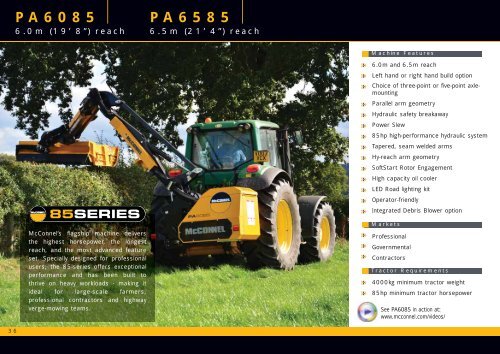The image is a color landscape-oriented photograph featured in an informational publication, depicting a tractor in a yard setting with a backdrop of grass and a tall tree. The tractor stands out with its bright yellow front and dark green enclosed driver's compartment. It has two large front wheels with yellow hubs and two smaller rear wheels. Prominently displayed on the front is the brand name "McConnell." Extending from the left side of the tractor is an arm attachment with a clipper mechanism, shown trimming the top of a hedgerow. The publication features a black strip across the top, highlighting the model numbers "PA 6085" and "PA 6585" in yellow, alongside technical dimensions in white text. On the right side, a white vertical rectangle with black text and bullet points details the tractor's features. The bottom left corner showcases a black panel with the "85 series" label, encompassing additional information about the tractor. The style combines photographic realism with graphic design elements.